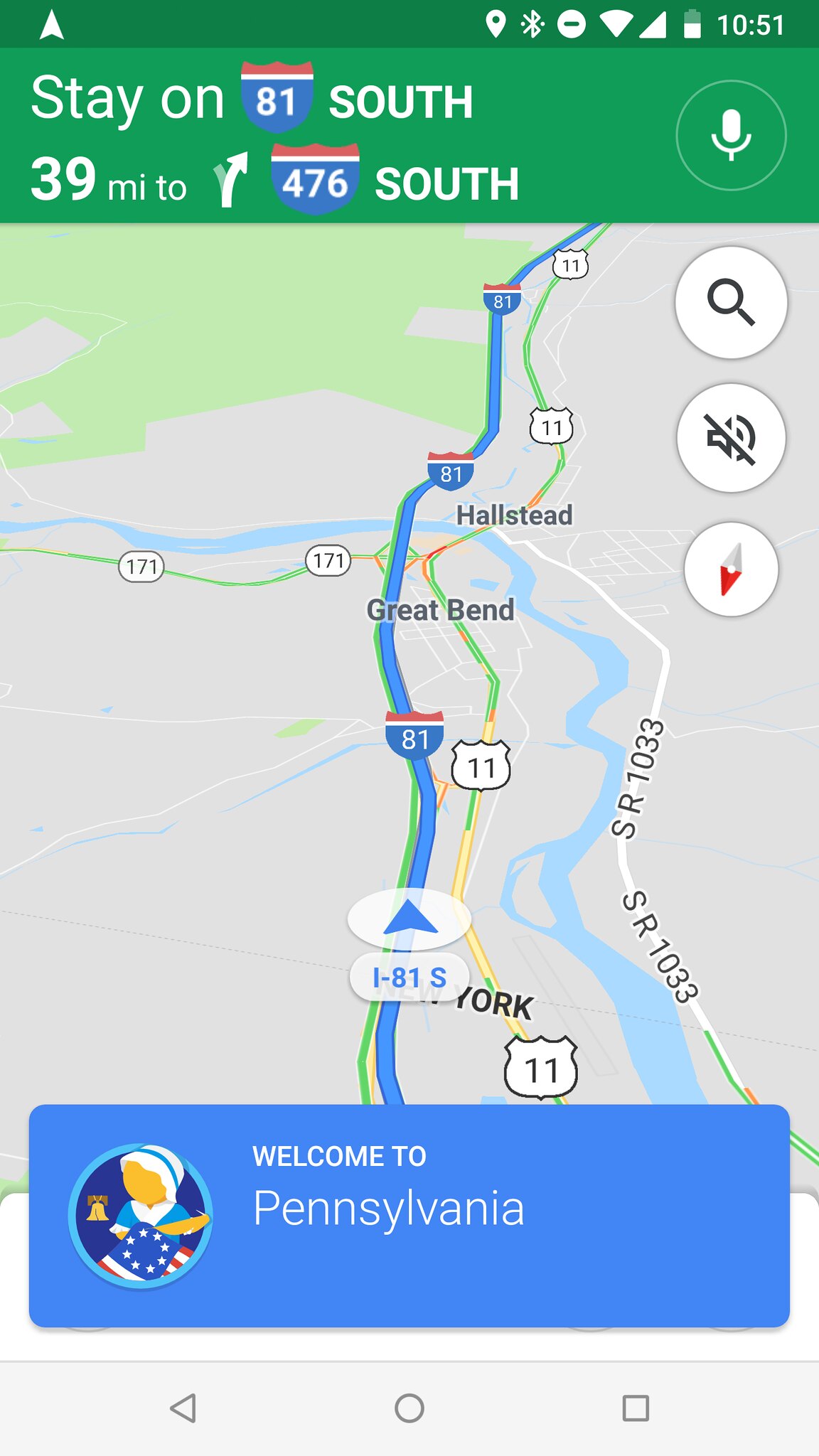A smartphone screenshot displays directions prominently. The topmost bar, dark green, shows the time as 10:51 on the right alongside various icons. Below, a larger bar with a green background and white text reads "Stay on 81 South," where "81" is depicted with a blue background and white and red stripes. Beneath this, it indicates "39 miles to" followed by a gently curving white arrow pointing right and the route "476 South." The bottom section of the screenshot features a detailed map. Highlighted in blue is the I-81 South highway, which stretches from a partially visible "York" at the bottom. Along the route, "Great Bend" is noted in the middle, with "Halstead" slightly further north on the right. The highway intersects Route 171 on the left and runs parallel to Route 11. At the very bottom, a blue band warmly welcomes, stating "Welcome to Pennsylvania."